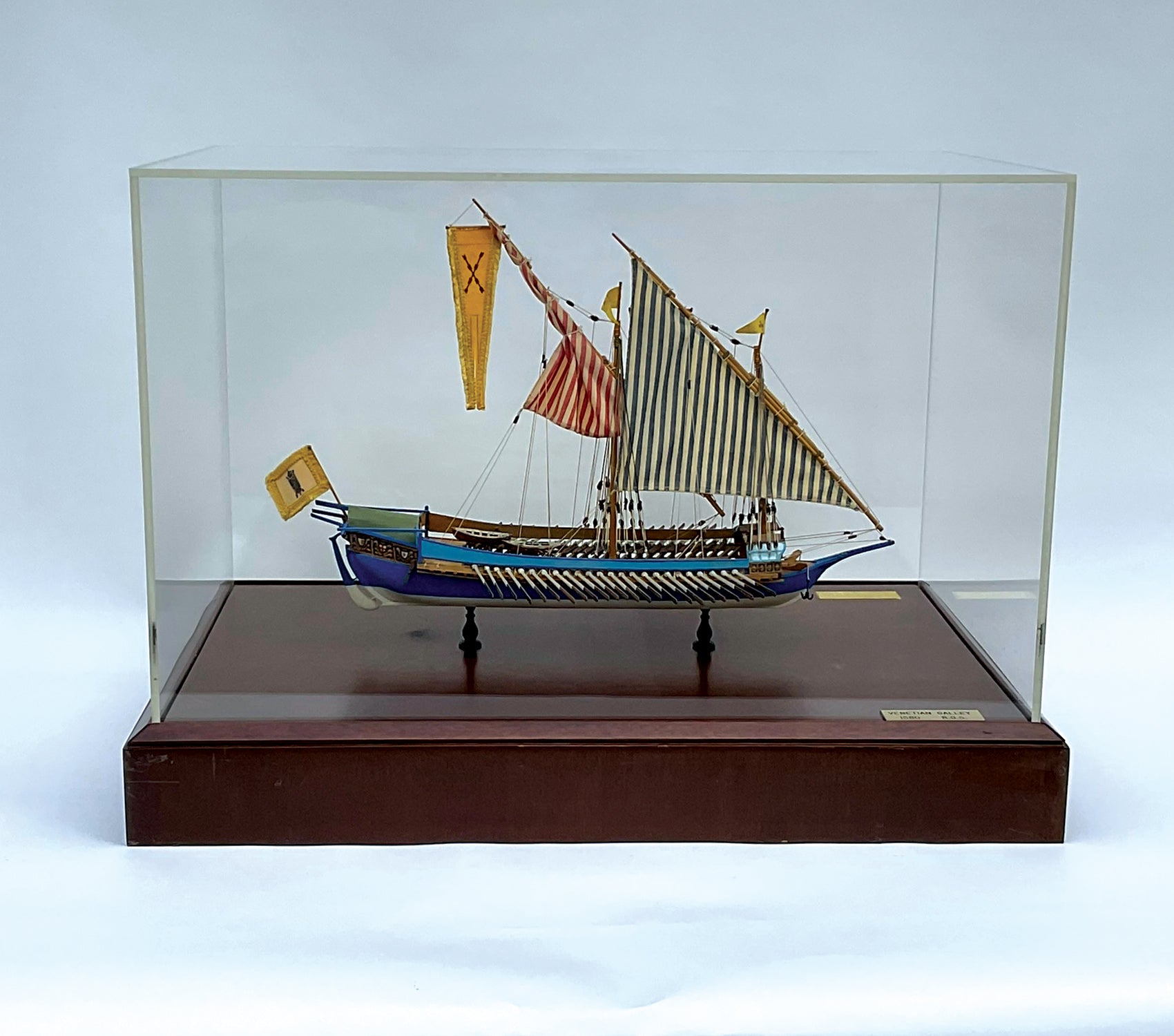This image depicts a meticulously crafted wooden model ship displayed in a museum-like setting inside a glass or acrylic case. The ship, evocative of ancient or historic vessels such as those from Viking or Egyptian times, is mounted on two prongs within the display. The base of the display case is a rich, dark wood, likely cherry or mahogany, adding to the elegance of the presentation.

On the deck of the ship, intricate details are visible, including two smaller lifeboats towards the stern. The hull features white slats and may have slots where oars once protruded, suggesting it is a rowing ship with a significant historical design. The ship boasts two sails: a fully extended black and white striped sail and a second sail that appears red and white striped, which is partially closed. Additionally, there are flags—one yellow with a black symbol extending from the stern, and another with an X at the end of the main sail with a yellow pennant.

The attention to detail in the model includes the ship's purple-blue painted base. The entire setup sits on a white surface with a white background, resembling an infinity wall, which helps highlight the ship’s striking features. A plaque is present on the base of the case but remains unreadable due to its angle. This display likely aims to represent the historical significance and craftsmanship of maritime vessels.